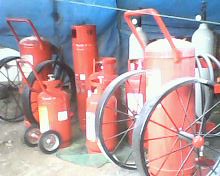The image depicts a scene with a blue canvas backdrop that occupies the entire background, complemented by a tan concrete floor. The main subjects are several orange tanks and barrels, some of which have white tops. These tanks vary in size, with some being short and others tall. Many of the tanks feature handles; the shorter ones have cylindrical shapes with handles at the top, designed for easy gripping and carrying, while the taller ones have rectangular handles that extend downwards, and are equipped with wheels for mobility. The wheels on the shorter barrels are small with rubber-coated, silver spokes, whereas the taller barrels have larger, all-metal wheels without rubber. In addition, two white canisters are visible at the back. Despite the image's blurriness, the array of wheeled and handled orange tanks against a blue canvas backdrop creates an industrial yet organized aesthetic.